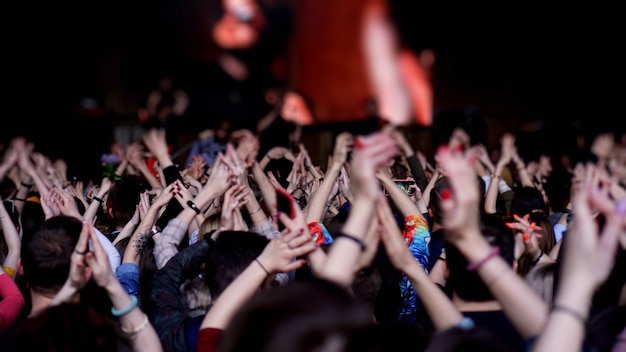The photograph captures a vibrant concert scene brimming with youthful energy. The main focus is the audience, a sea of younger people with their hands raised high in a distinctive triangular gesture, fingertips touching and elbows spread apart. Their raised arms dominate the picture, obscuring faces and upper bodies, suggesting the photo was taken in the midst of enthusiastic clapping or movement. The crowd is primarily dressed in dark attire, punctuated by splashes of color – notably, one individual stands out with a bright blue and red tie-dye top. Various hands are adorned with colorful bracelets and painted nails, adding a touch of personal flair. The background is a blur, with the stage only hinted at by a reddish glow and indistinct lights, directing the focus firmly on the animated audience. The overall scene exudes a sense of collective celebration and excitement, typical of a lively indoor concert.